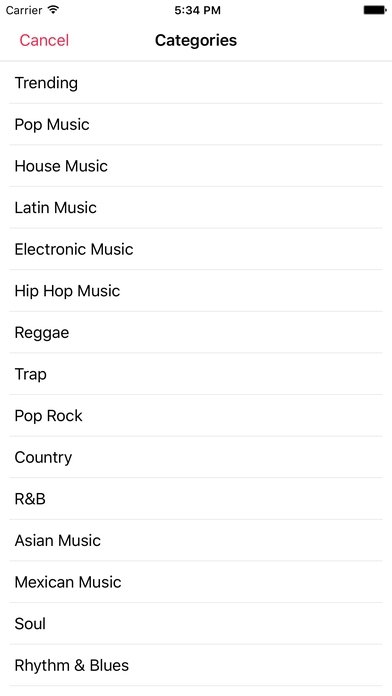**Descriptive Caption:**

A clear screenshot of the category section on the Apple Music app, displayed on a cell phone with a white background. Prominently at the top left in purple font is the word "Cancel." Centered at the top of the page, the title "Categories" is displayed in bold black font. Below, a vertically arranged list of music categories includes: Trending, Pop Music, House Music, Latin Music, Electronic Music, Hip Hop Music, Reggae, Trap, Pop Rock, Country, R&B, Asian Music, Mexican Music, Soul, and Rhythm and Blues. Each category is separated by a thin gray line, resembling lined paper toward the right side due to the empty white space. 

In the status bar at the top left corner, “Carrier” is displayed in small black letters, followed by a Wi-Fi icon. The current time is centered at the top, and on the far right, a full battery icon is visible.